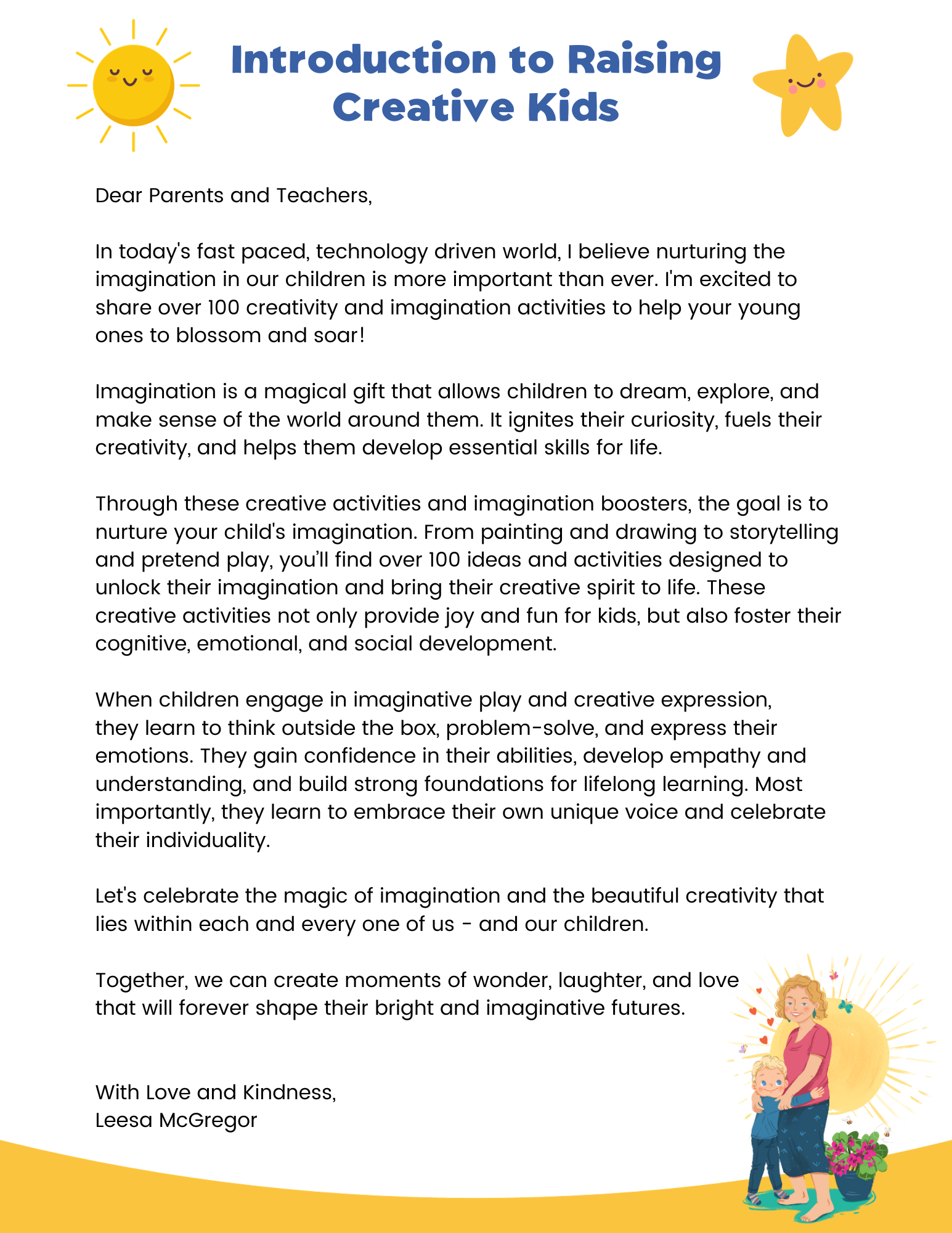This is a single-page pamphlet titled "Introduction to Raising Creative Kids," prominently displayed in blue text, with "Introduction to Raising" at the top and "Creative Kids" just below it. The design features cheerful illustrations of a smiling sun on the left and a smiling star on the right, both in yellow. The main text begins with "Dear Parents and Teachers," highlighting the importance of nurturing imagination in children in today's fast-paced, technology-driven world. The pamphlet enthusiastically promotes over 100 creative and imagination-boosting activities aimed at helping children blossom and soar.

The text explains that imagination is a magical gift that enables children to dream, explore, and understand their world. These activities, ranging from painting and drawing to storytelling and pretend play, are designed to unlock creativity and foster cognitive, emotional, and social development. Engaging in these activities helps children think outside the box, solve problems, express emotions, build confidence, develop empathy, and celebrate their individuality. The message concludes with an invitation to celebrate the magic of imagination and the beautiful creativity in every child.

At the bottom, there's a yellow stripe, and on the lower right corner, an illustration of a mother and child with a sun and a flowering plant adds a heartfelt touch. The pamphlet is signed, "With love and kindness, Lisa McGregor." 

The colors throughout include yellows, pinks, dark blue, brownish tones, orange, pale yellow, pale red, pale blue, and blonde, enriching the inviting and vibrant design.